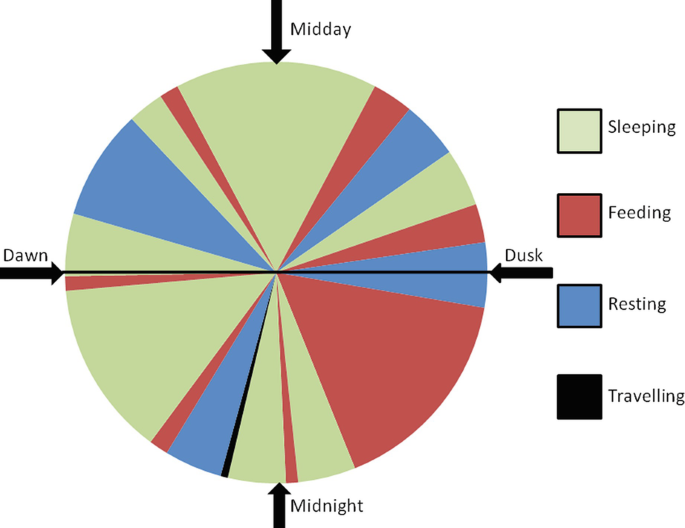The image is of a circular pie chart divided into various colored slices, each representing a different activity and time of day. The chart includes a key for the colors and labels for the times. The light green sections, which denote sleeping, are the largest, with one prominent slice at the top labeled "midday" and smaller green slices distributed throughout. The dark red slices, representing feeding, are predominantly grouped in a significant portion at the lower right corner, with several smaller slices interspersed. The blue slices, indicating resting, are smaller and scattered across the chart. The black slices, the smallest, symbolize traveling. Arrows point to specific slices, marking the times of day—midday at the top (12 o'clock), dusk at the right (3 o'clock), midnight at the bottom (6 o'clock), and dawn at the left (9 o'clock).